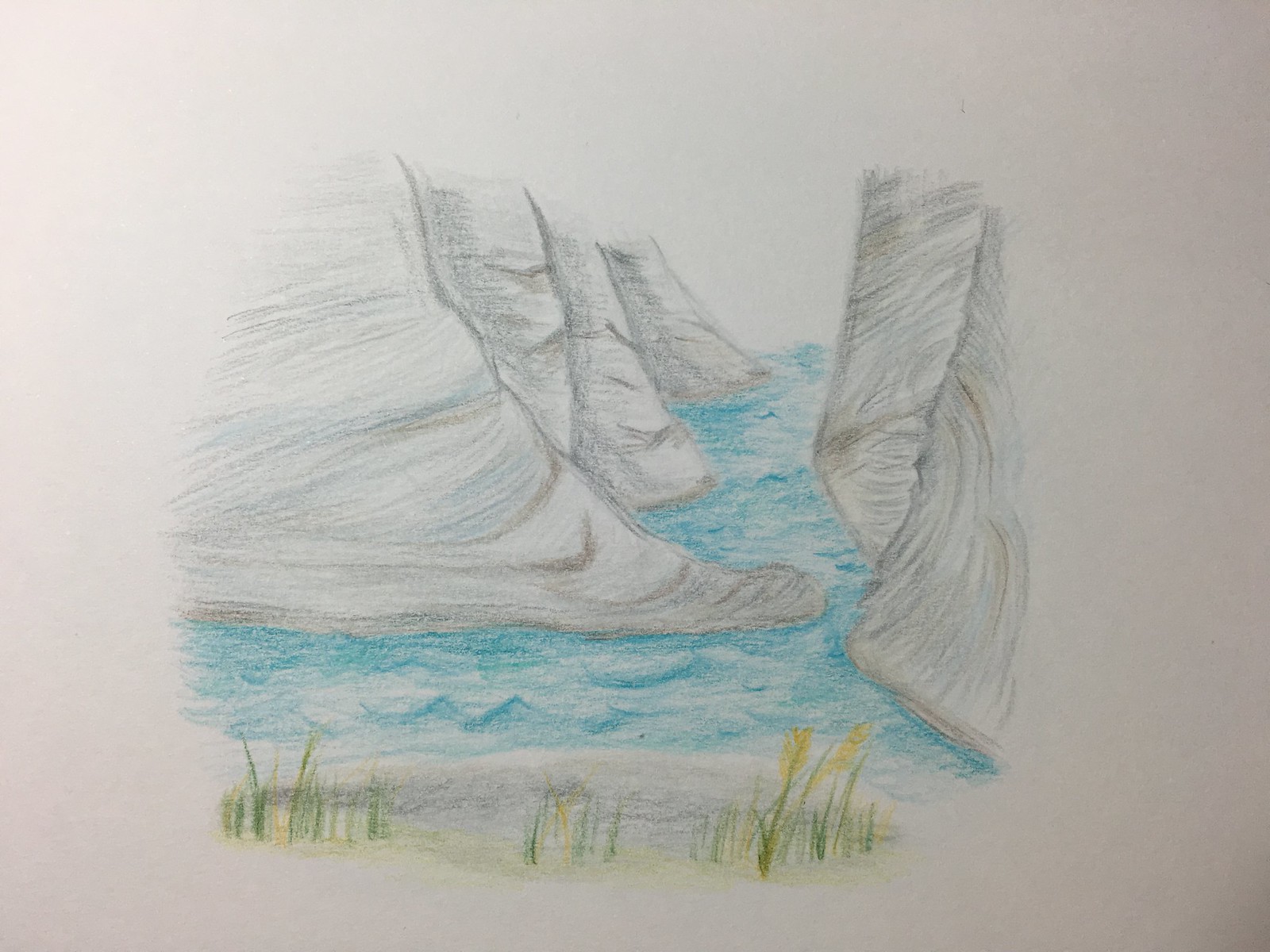This evocative artwork portrays a serene river winding through a dramatic gorge. Using shades of gray to black, the artist skillfully depicts rugged mountainsides, providing a stark contrast to the vibrant blue waters that flow between them. The river's surface is accented with blue waves and deeper blue reflections, suggesting movement and depth, likely created with Crayola-based mediums. On the banks of the river, patches of lush green grass transition into golden hues, hinting at a sunlit afternoon. Additionally, some of the plants exhibit green leaves with golden tips, enhancing the scene's rich and varied palette. The drawing, set against a pristine white paper background, brings together natural elements in a compelling and picturesque landscape.